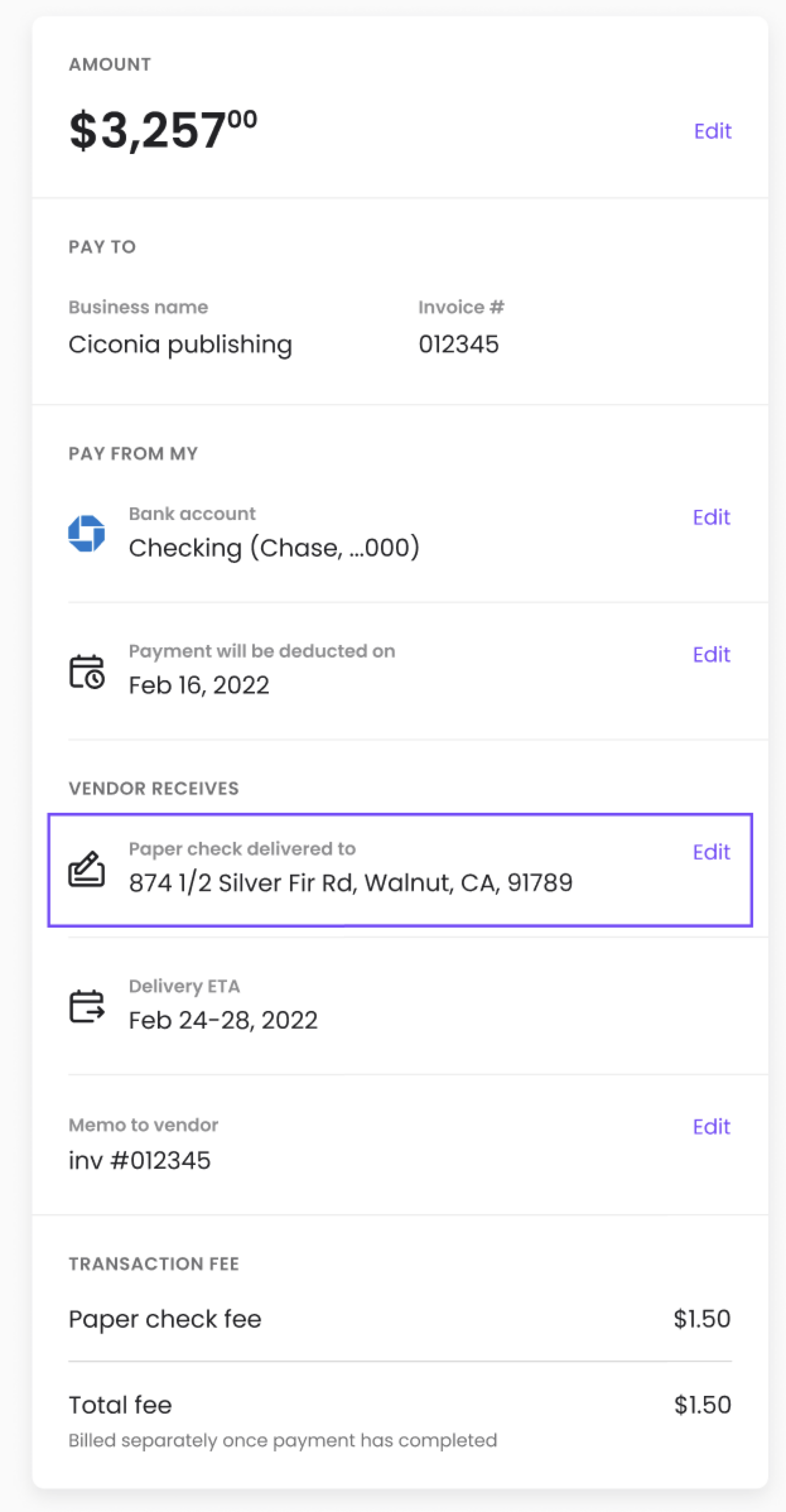The image displays an invoice amount, likely as an overlay on a smartphone screen. In the top left corner, a large bold black text shows the amount due of $3,200, along with an additional charge of $257.00. Just below this, the text "P2" is written in gray.

The business name "Ciccone Publishing" appears prominently followed by "Invoice 012-345." Directly underneath, it specifies that the payment will come from a checking account with Chase bank, labeled as "Pay for my bank account checking Chase (delta bill 00)." To the right of this information is an "Edit" option.

Further down, it states: "Payment will be deducted on February 16, 2022." Below this, a note mentions that a paper check is scheduled to be delivered to "874 Have Solar for a Road, Walnut, California, 91789," with an estimated delivery date of "February 24, 2022."

Additionally, the memo for the vendor reads "Invoice number 012-345," and this section also includes an "Edit" button. A "Transaction Fee" section in gray follows, detailing a "Paper Check Fee: $1.50" and a "Total Fee: $1.50." It is noted that the total fee will be billed separately once the payment is completed.

A blue box highlights the section containing the delivery information for the paper check.